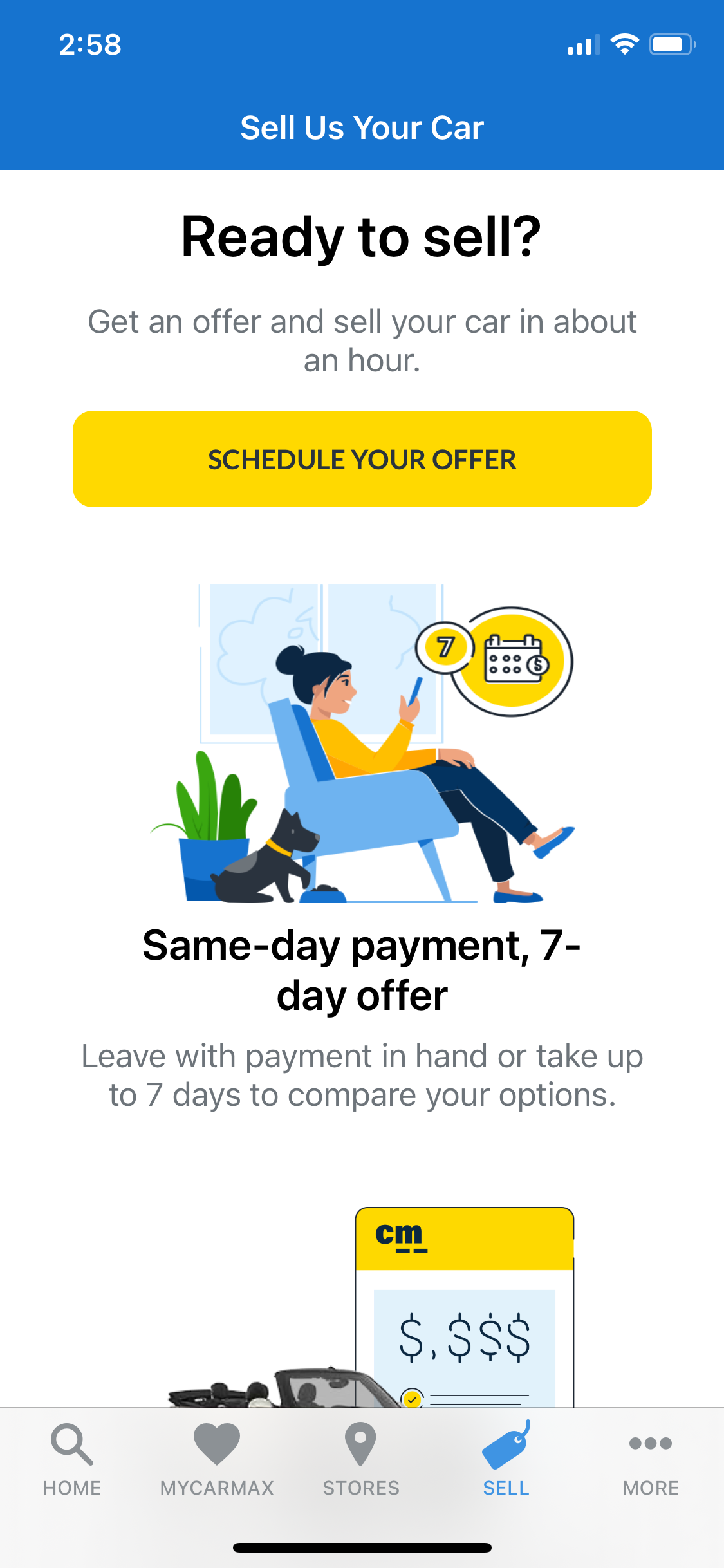The image is a small, mobile-friendly representation of a website designed for selling cars. At the top of the phone screen, there is a blue band displaying white text that reads "2:58," without specifying AM or PM. The status bar also shows typical phone indicators: signal strength, Wi-Fi connectivity, and a nearly full battery.

Below the blue band, the main content area begins with a bold headline on a white background reading "Sell Us Your Car." Underneath, in large letters, it says "Ready to Sell?" followed by a subheading, "Get an offer and sell your car in about an hour." 

A prominent yellow button beneath this subtext says "Schedule Your Offer." The middle section of the image displays an illustrated woman with dark hair in a bun, wearing a yellow shirt, blue pants, and blue shoes, seated in a blue chair in front of a window. She is holding a phone, and her phone screen shows a calendar. A plant is positioned behind her chair, and a dog sits next to her. 

The illustration is accompanied by text stating, "Same day payment, 7 day offer. Leave with payment in hand or take up to 7 days to compare your options." At the bottom, another yellow bar features the initials "CM," likely representing CarMax.